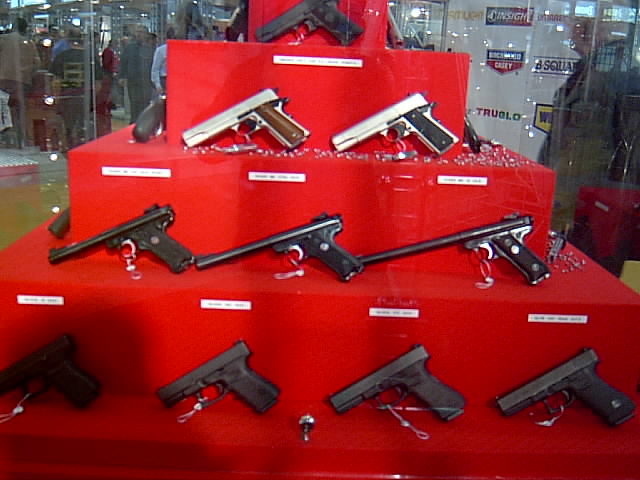The image depicts a vibrant red, tiered pyramid-like display, resembling a multi-layered wedding cake, showcasing an array of firearms within a store setting. The display comprises four levels. On the bottom tier, there are four black handguns. The second tier features three handguns with notably long barrels, likely older models. Ascending to the third tier, two silver handguns are displayed; the one on the left boasts a brown wooden handle, while the one on the right has a black handle. Crowning the top tier is a solitary black handgun.

The background showcases a glass partition with various company logos, including "True Glow." The glass structure provides a view of several individuals outside the partition, among them an older person with white hair in a black jacket, and a few men, including one in a brown sweatshirt and pants, and a balding man in a black shirt with blue pants. The setting, with its meticulous arrangement and notable onlookers, suggests the possibility of a gun show.